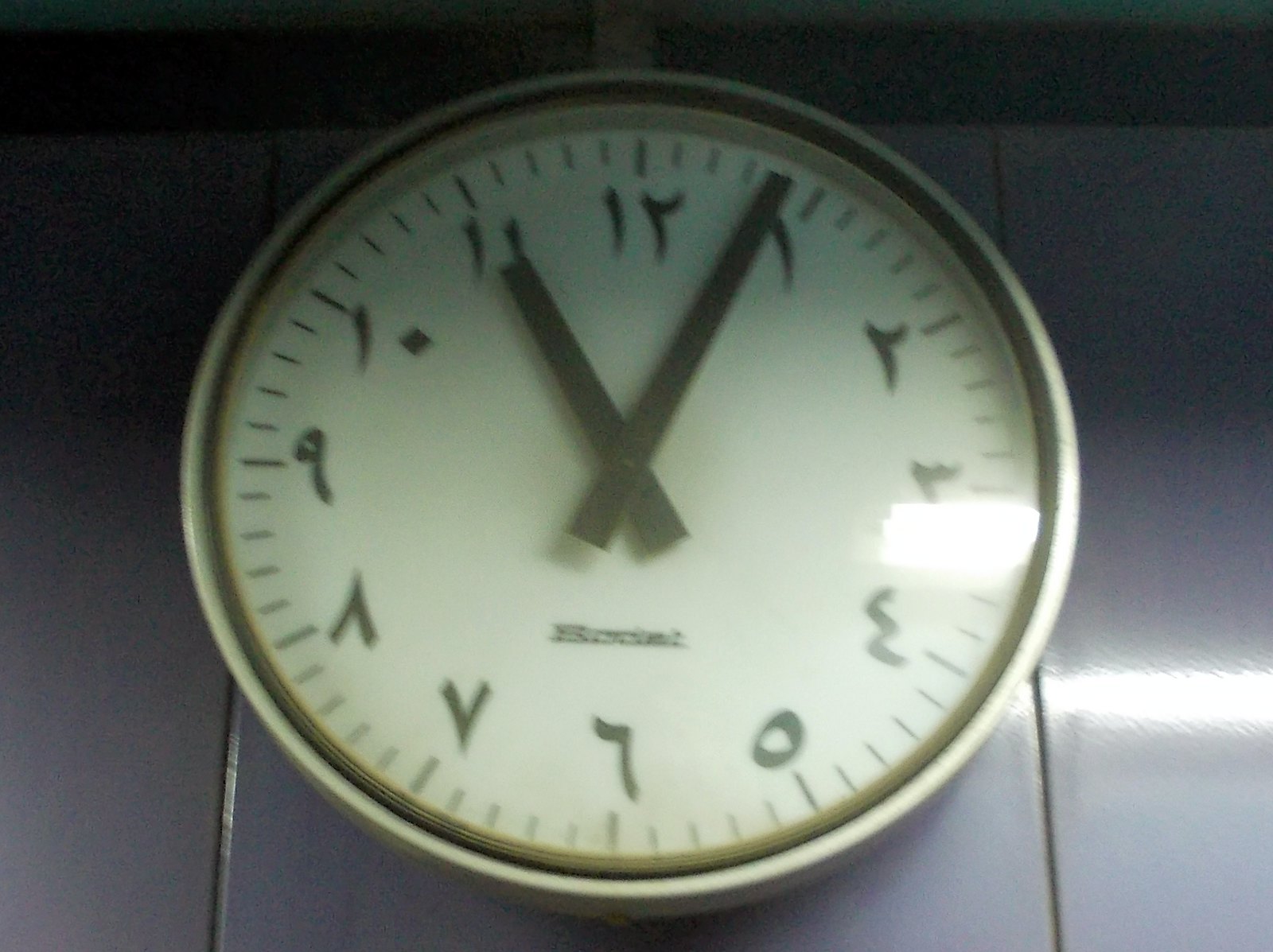This is a close-up image of an unusual white-faced wall clock mounted on a gray paneled or wooden wall. The clock features a creamy white face encased in a silver band, with a glass cover adding a reflective sheen. The numbers on the clock face are notably unconventional, displaying a mix of Hebrew characters and distorted digits, with some appearing backwards or misplaced. For example, the number three is reversed, and the number nine is one of the few correctly placed digits. The clock is showing the time at approximately 11:04. The hour and minute hands are black and crafted from metal, contributing to the clock's sleek, modern appearance. The structure to which the clock is attached is also made of metal and painted gray, complementing the overall aesthetic.